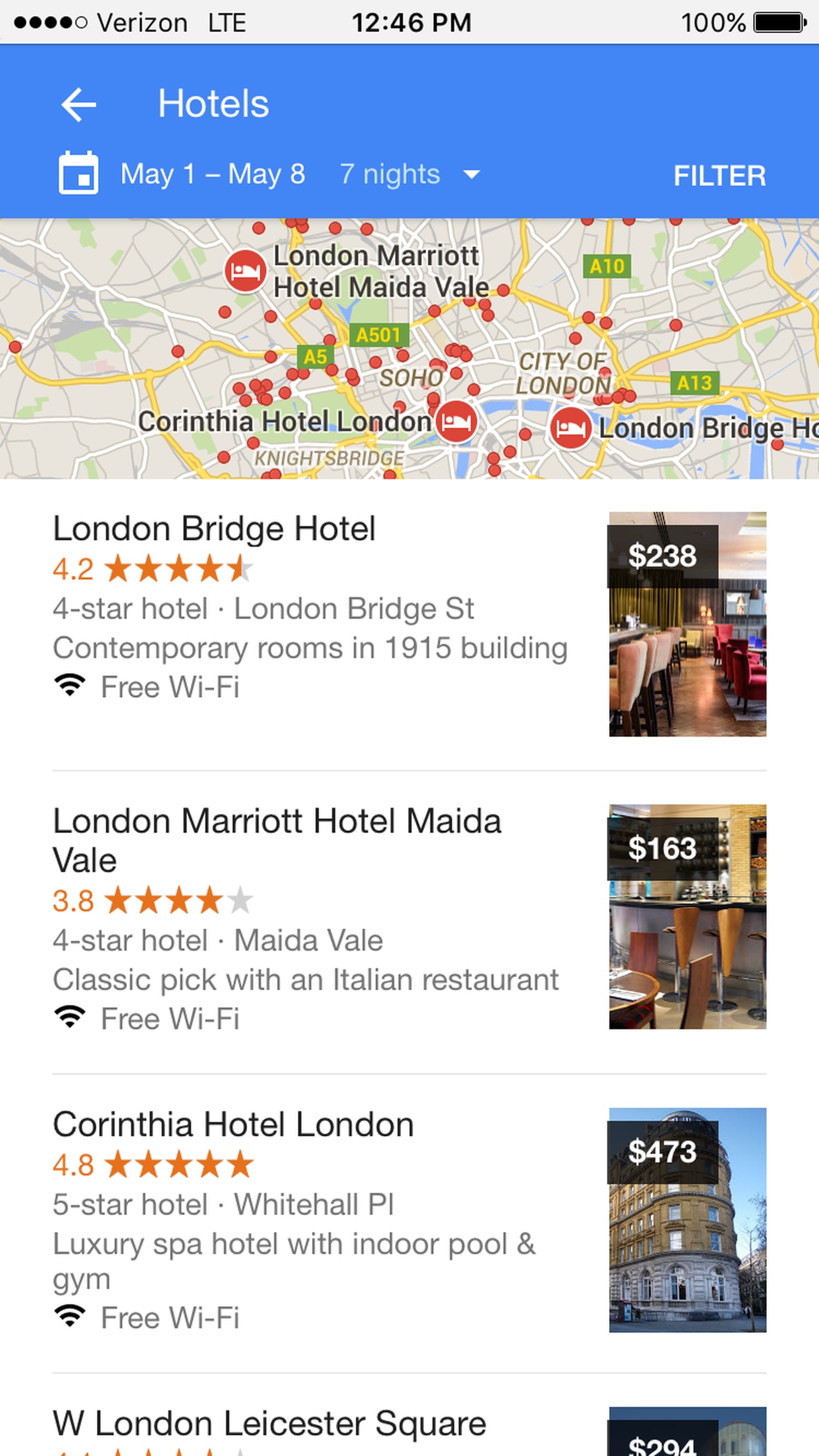A digitally-rendered image showcases a hotel booking interface designed for a mobile device. At the top of the screen, the word "Hotels" is prominently displayed. Directly below this, the dates "May 1st through May 8th" are listed, accompanied by a small white calendar icon, indicating a booking period of seven nights. To the right, a white "Filter" button is visible.

In the center of the screen is a detailed map of London, marked with various points of interest. Key locations such as Soho, the City of London, and Knightsbridge are highlighted. Red bed icons signify hotel locations, while green markers labeled with alphanumeric codes (e.g., A5, A10, A13) are also present. The map is detailed with yellow, white, and gray lines representing different roads.

Below the map, a list of hotel options is provided:

1. **London Bridge Hotel**: Priced at $238 per night, this four-star establishment has a 4.2-star rating. It features contemporary rooms in a historic 1915 building and offers free Wi-Fi.
   
2. **London Marriott Hotel Mayfair**: This hotel is rated 3.8 stars and costs $163 per night.
   
3. **Corinthia Hotel London**: A luxurious option priced at $473 per night.
   
4. **700 London Leicester Square**: Mid-range pricing at $294 per night.

Each listing includes essential details such as the hotel's name, rating, price, and a brief description.